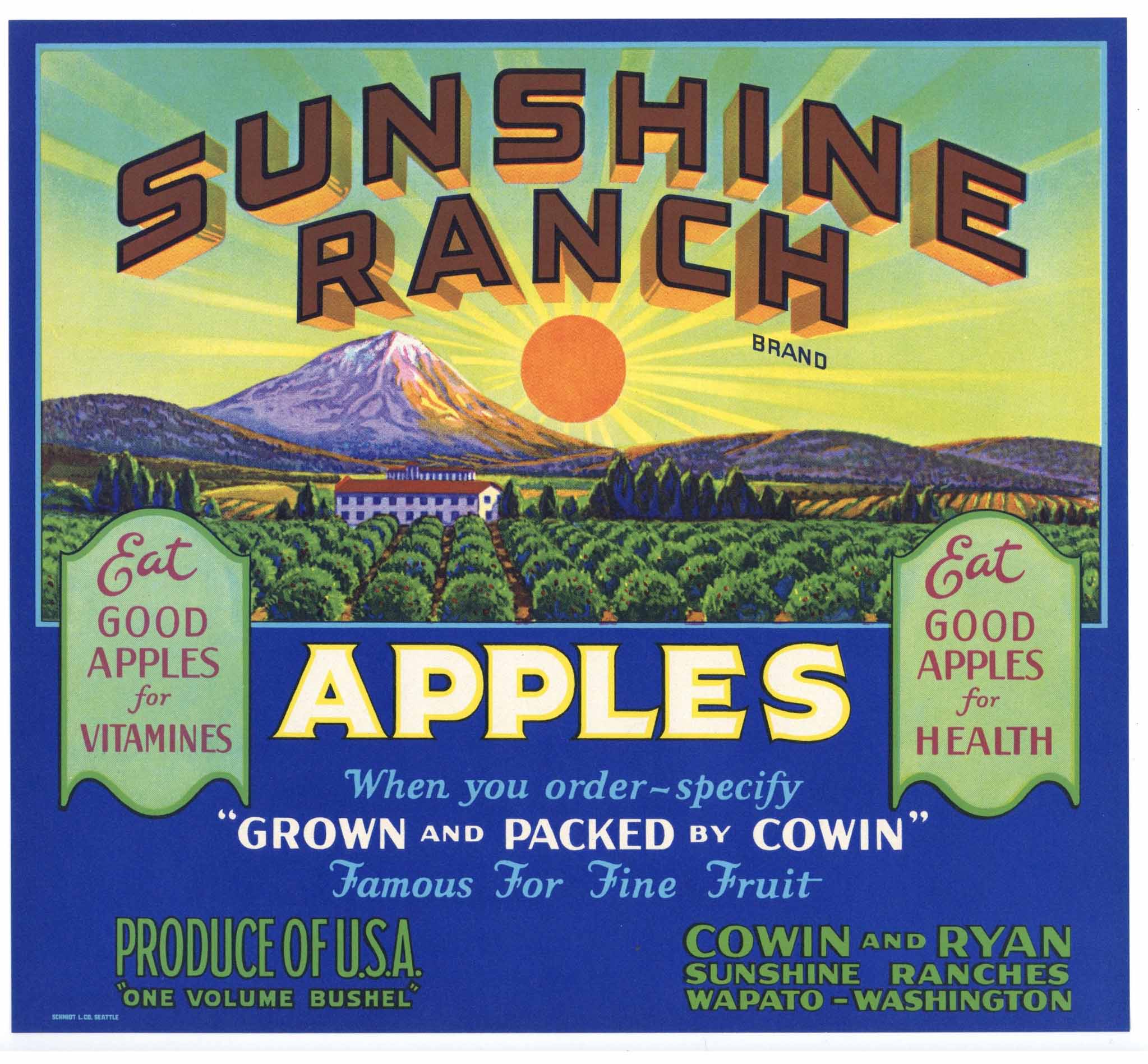The promotional poster for Sunshine Ranch Brand has a bold, captivating blue background. At the top of the poster, "Sunshine Ranch Brand" is prominently displayed in bold, 3D brown lettering. Below this, an illustration showcases an orange sun with vibrant yellow rays extending outward, rising over a snow-capped mountain range. Nestled beneath the mountains, a sprawling ranch with meticulously aligned rows of bushes leads up to a two-story white mansion with a red roof and multiple windows. To the left, a green panel declares, "Eat Good Apples for Vitamins," mirrored by another green panel to the right that says, "Eat Good Apples for Health." The center text, in eye-catching yellow print, simply reads, "Apples." Scattered across the bottom of the blue background, the text informs potential customers, "When you order, specify grown and packed by Cohen. Famous for fine fruit. Produce of U.S. One volume bushel. Cohen and Ryan Sunshine Ranches, Wapato, Washington." This detailed and colorful illustration captures the essence of natural, wholesome fruit cultivated with care at the Sunshine Ranch.